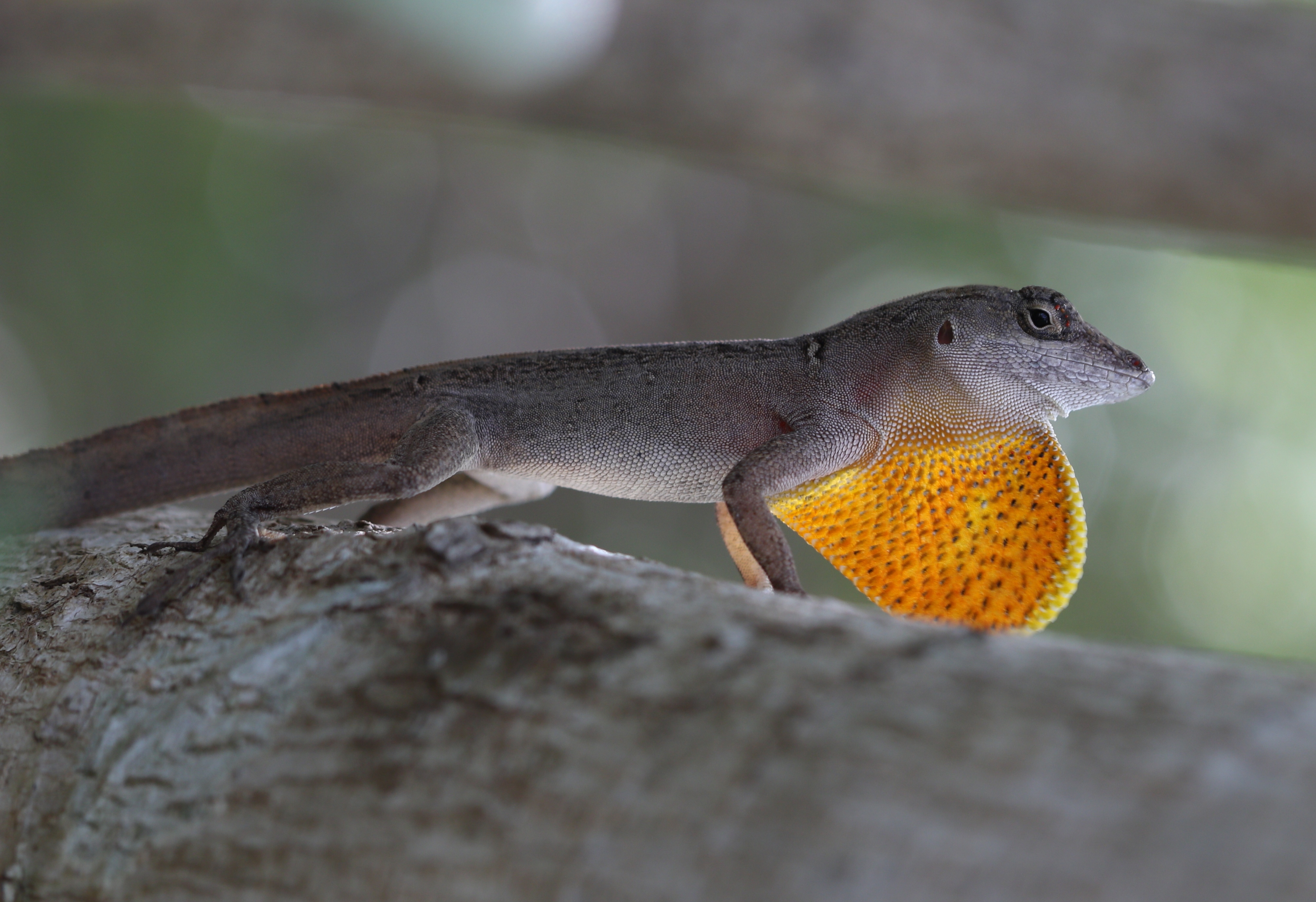A detailed close-up shot captures the side profile of a small, thin lizard standing on a large, gray tree branch, blending almost seamlessly with its surroundings due to its similarly gray-hued skin. The lizard is poised still, its slightly disproportionately larger head in line with its long, thin body and equally thin legs. A striking feature is a bright yellow, oval-shaped flare extending from beneath its chin, dotted with small black spots—reminiscent of a defensive or display mechanism similar to a frog's inflated throat sac. The image background is a blurred mix of green and gray tones, suggesting a natural, vegetative setting. The focus gradually sharpens from the bottom right to the left, emphasizing the gray tree branch on which the lizard's tail extends, disappearing out of frame. The lizard’s eye is open, appearing to gaze directly at the camera, with a small black dot visible behind it, marking an ear hole. This vivid yellow flare against the muted gray palette makes for a visually striking contrast in the composition.